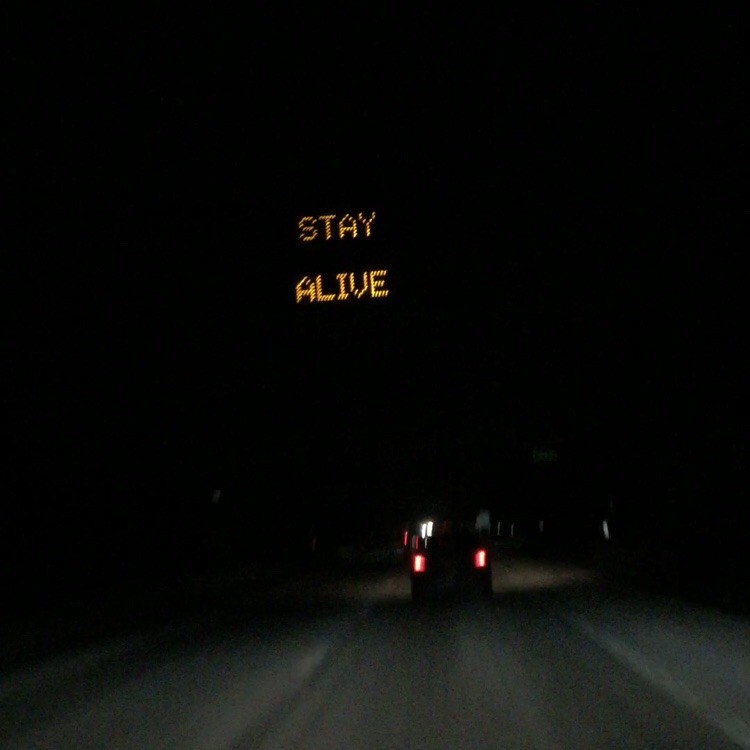In this point-of-view night shot from inside a car, we see a dimly lit two-lane highway. The photograph captures a particularly dark stretch of road, where the only visible elements are illuminated by car headlights. Ahead, a black car with red taillights can be seen, providing some light in the otherwise pitch-black environment. The road itself is dark asphalt, with barely discernible white lines on the right and dotted lines in the center. An overhead digital sign, characterized by its orange-yellow illuminated text, reads "Stay Alive." The sign's programmable nature suggests it can display various messages, but at this moment, it serves as a reminder for safety on this poorly lit and treacherous night drive. The extremely low visibility emphasizes the importance of the sign’s message.